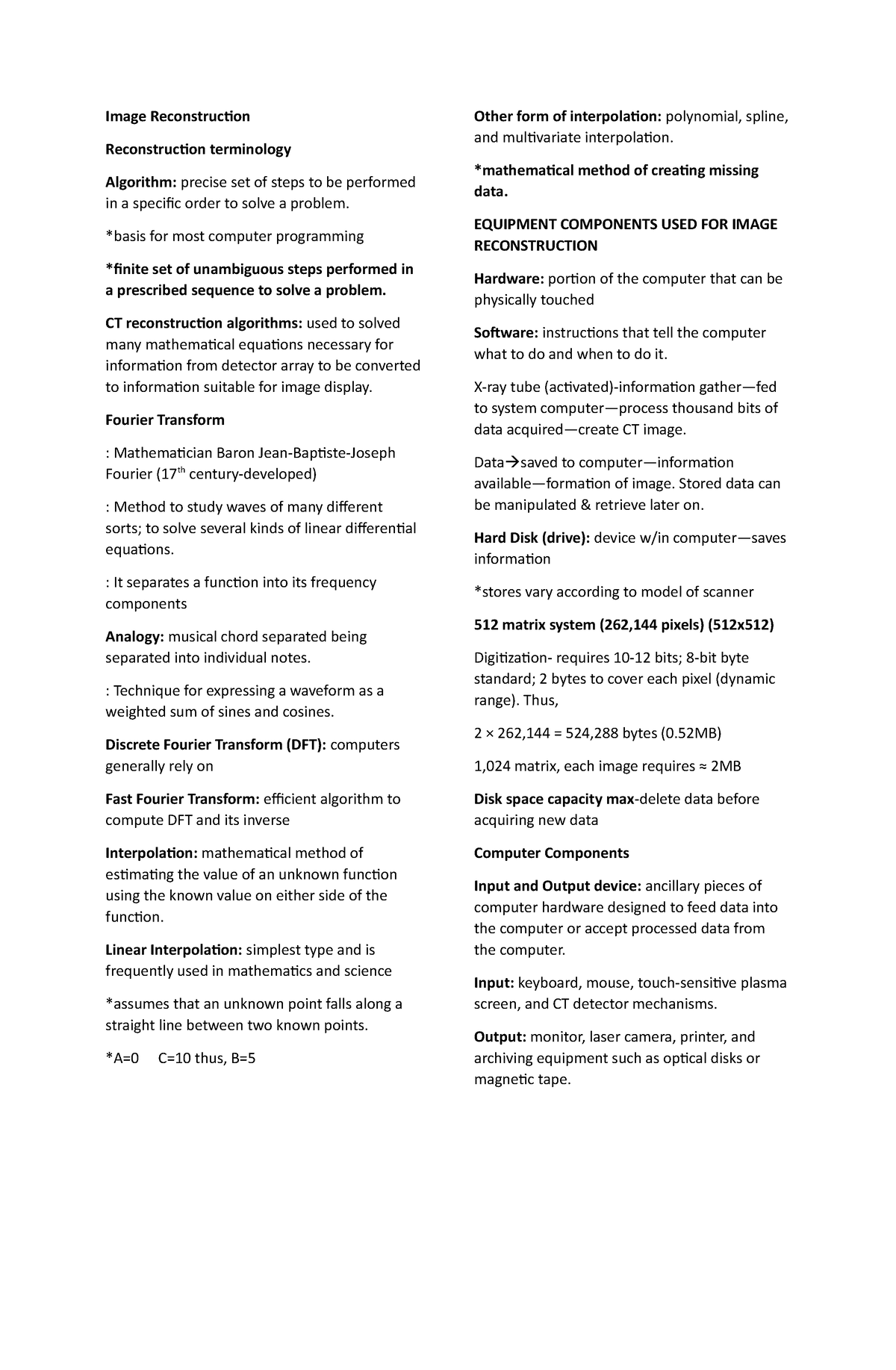A detailed descriptive caption for the image could be:

"This image showcases an in-depth explanation of image reconstruction terminology and algorithms. It highlights the precise set of steps, or algorithms, essential for solving problems, which form the foundation of most computer programming. The image provides a comprehensive description of these steps being finite and unambiguous, performed in a prescribed sequence. Specifically, the caption delves into CT (Computed Tomography) reconstruction algorithms, explaining their importance in solving various mathematical equations to convert data from a detector array into suitable information for image display. An analogy is provided, likening the process to separating musical chords into individual notes. The image also outlines the hardware and software components crucial for image reconstruction. Hardware refers to the physical parts of the computer, while software comprises the instructions that guide the computer's operations. Mention is made of the hard disk drive, the device within a computer that saves information, and emphasizes the importance of managing disk space capacity by deleting old data before acquiring new data."